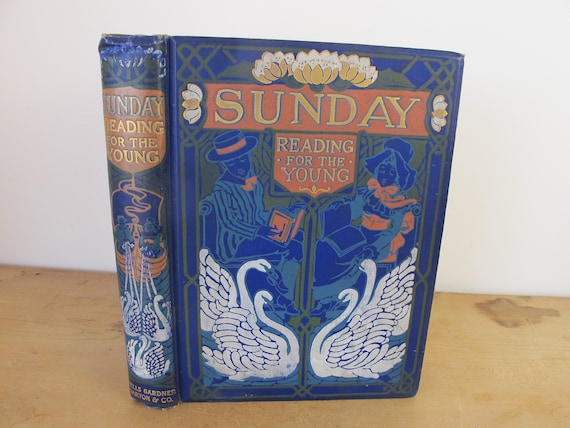The image depicts a color photograph of an old hardcover book, standing upright on a light wooden surface against a white wall. The book's cover and spine are predominantly indigo blue. On the spine, a reddish shield displays the title "Sunday Reading for the Young" in gold lettering, beneath which are four white swans and a group of people in a boat.

The front cover features an intricate design with white and yellow flowers forming an arch at the top, flanking a red banner with the word "Sunday" in gold, outlined in blue. Below this banner is another red rectangle with "Reading for the Young" inscribed in gold. On either side, there are silhouettes of a man and a woman: the man on the left is depicted in a striped blazer and boater's hat, holding a book, and he has accents of orange on his bow tie and hat ribbon. The woman on the right is dressed in a frilly gown with a bonnet, and has orange accents on the bow at her neck and her belt. At their feet, four white swans are arranged in a serene formation.

This visually vibrant book cover, combining rich colors and detailed imagery, stands out on the simple wooden surface with the plain white wall providing a minimalist backdrop.